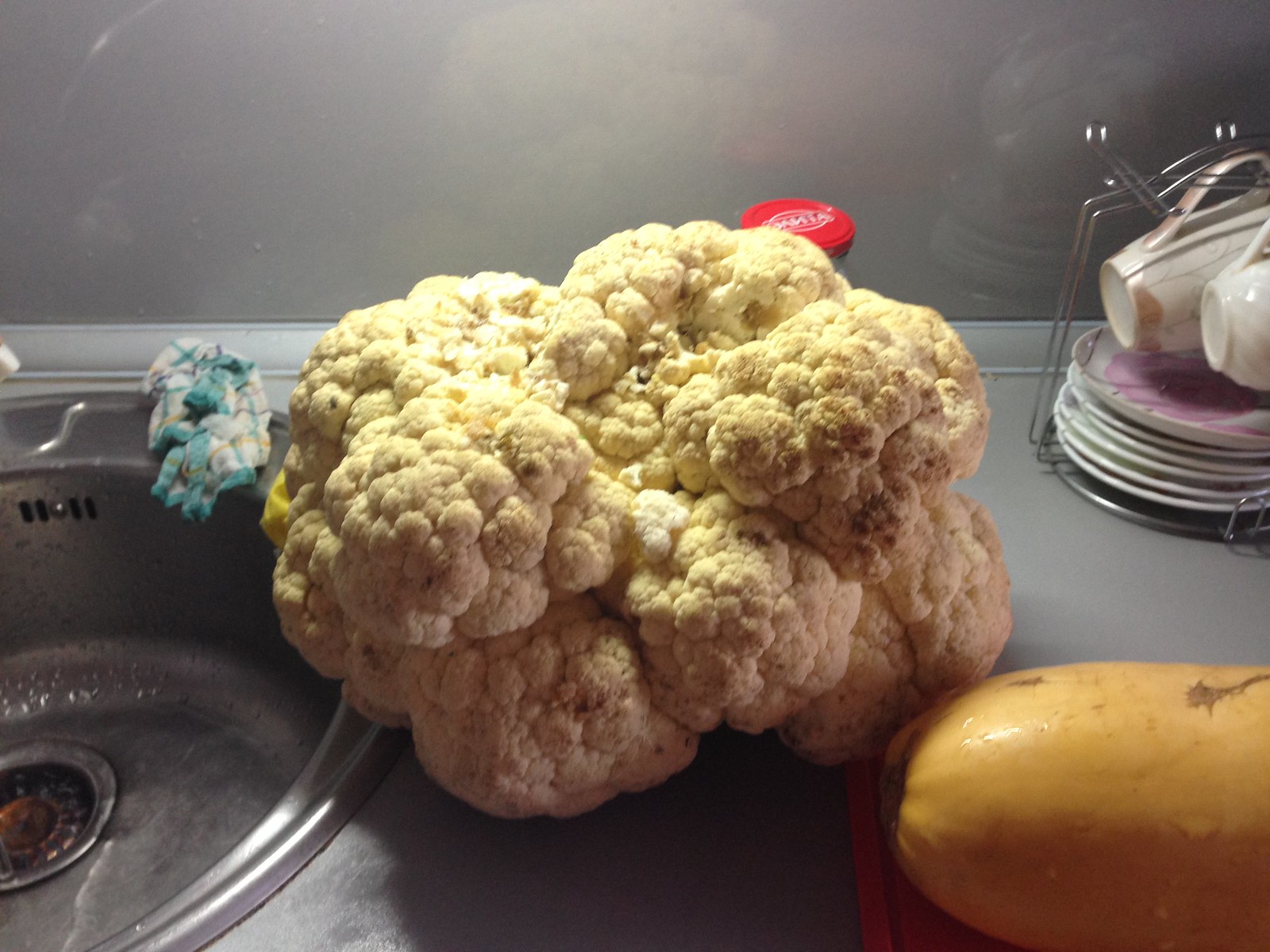This detailed photograph captures a kitchen countertop scene. On the left side of the image, a large, white cauliflower bunch, slightly dirty and awaiting washing, sits prominently next to a round sink. The sink, which has visible water spots, features a green, blue, and white washcloth with blue and yellow stripes draped over its edge.

Just to the right of the cauliflower, there is a butternut squash with a small brown spot, resting on a red surface. Behind the cauliflower is what appears to be the red lid of a jar, partially obscured with white writing on top. Further to the right, a metal rack holds a collection of teacups and coffee saucers, with what looks like six small plates neatly arranged beneath them on the gray, slightly shiny countertop. The background reveals a gray wall, transitioning into a darker gray accent with a light trim.